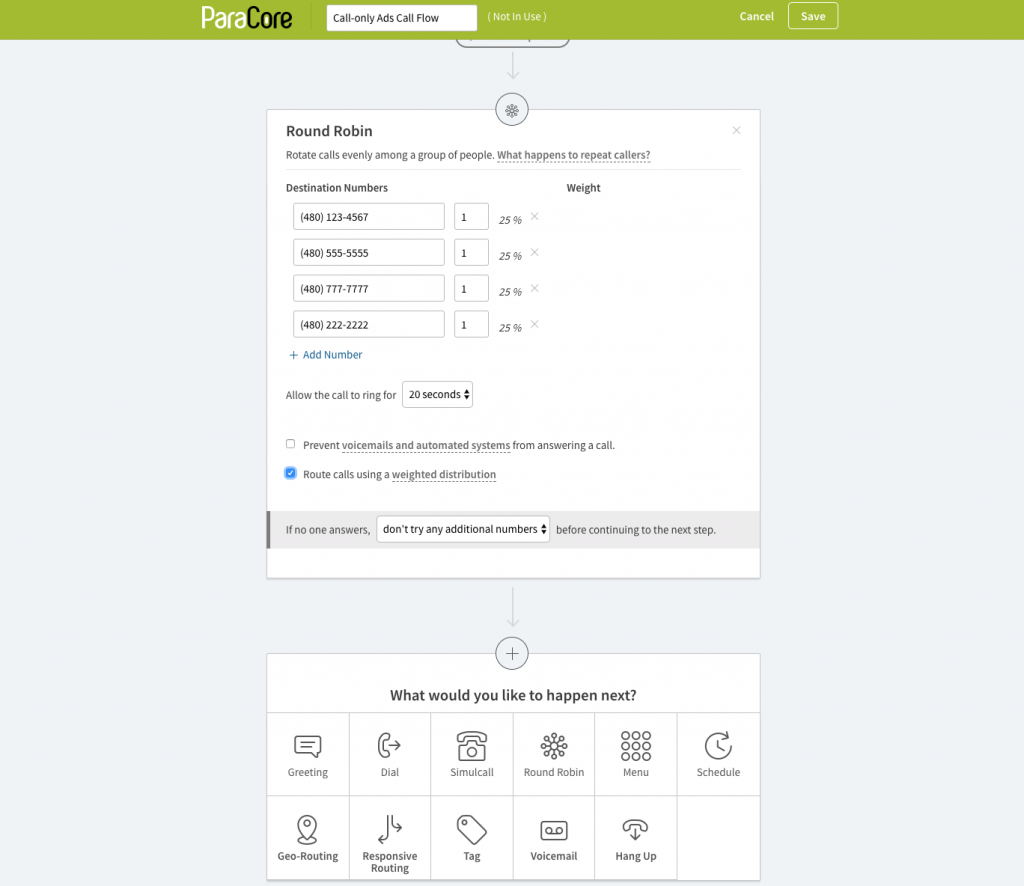Screenshot of a website showcasing a call management interface for ParaCore, a company or service name highlighted in a light green banner at the top of the page. The banner prominently displays "ParaCore" in bold letters. Underneath the banner is a white box with call settings options labeled "Call only adds call flow, not in use," alongside "Cancel" and "Save" buttons.

The central part of the screen addresses how incoming calls are routed, suggesting options to "Rotate calls evenly among a group of people" and inquiring, "What happens to repeat callers?" The default setting appears to be "Round Robin." Detailed under this are four destination numbers:
1. 480-123-4567 with a weight of 25%
2. 480-555-5555 with a weight of 25%
3. 480-777-7777 with a weight of 25%
4. 480-222-2222 with a weight of 25%.

A button labeled "Plus, add number" allows for the addition of more numbers. 

Other settings include instructions to allow calls to ring for 20 seconds, prevent voicemails and automated systems from answering, and route calls using a weighted distribution. There is also a stipulation that if no one answers, the system should not try additional numbers before continuing to the next step.

The interface then asks, "What would you like to happen next?" and presents several options: Greeting, Dial, SimulCall, Round Robin, Menu, Schedule, Georouting, Responsive Routing, Tag, Voicemail, and Hang Up.